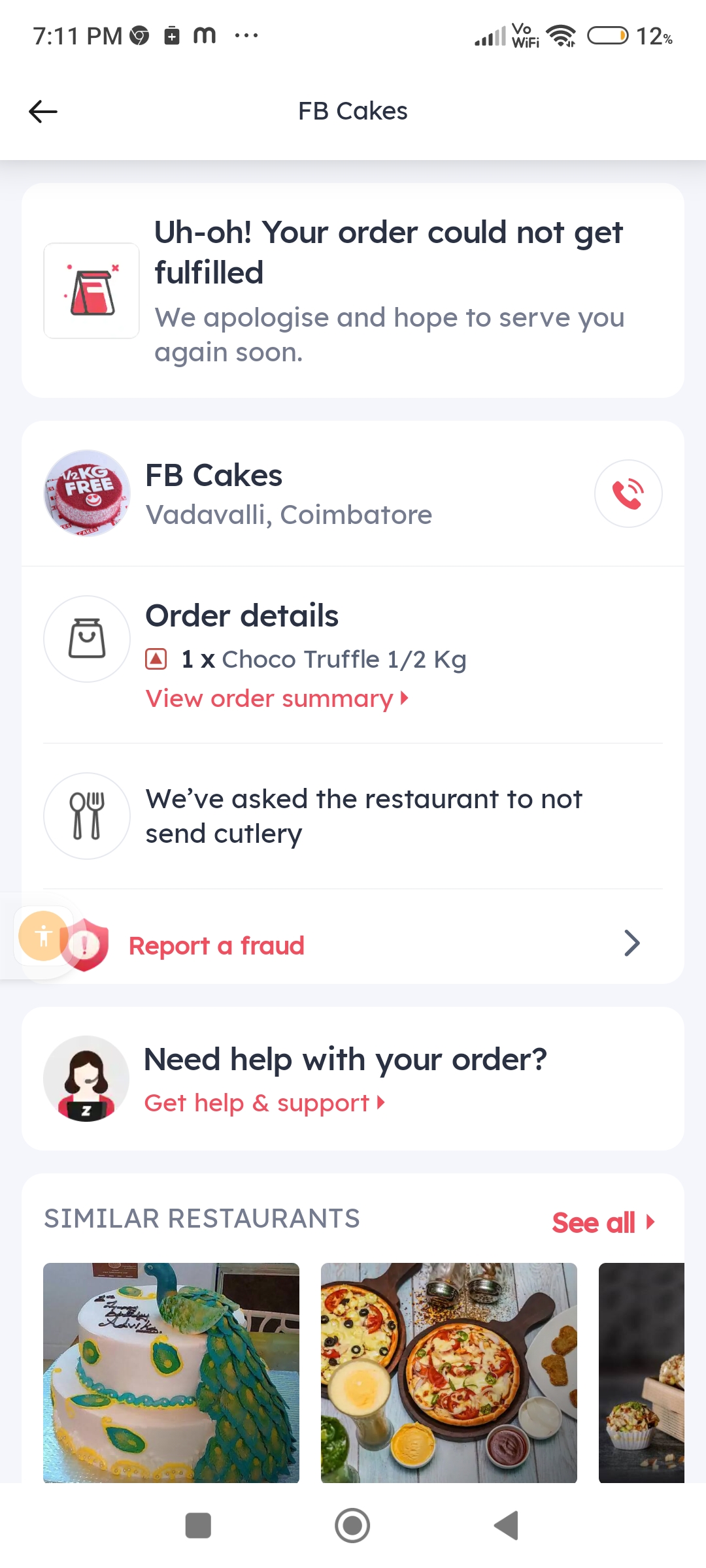The image is a rectangular screenshot of a cake ordering page from a mobile device. In the upper left corner, a timestamp reads "7-11 p.m." On the upper right, a battery indicator, outlined in dark gray, shows a low battery level at 12%, highlighted by a small sliver of dark orange.

Central to the image is the page title, "F.B. Cakes," situated toward the top. Below the title, a prominent error message is displayed, featuring a small red paper bag icon on the left. The message in black text states, "Uh oh, your order cannot get fulfilled." Directly beneath this, a light gray text offers an apology: "We apologize and hope to serve you again soon."

Further down, additional information about the company is provided. The heading "F.B. Cakes" is followed by the company's address. Below that, in bold black text, "Order Details" is listed. Included in this section is a notification reading, "We've asked the restaurant to not send cutlery."

At the bottom of the page are options for further assistance, including a "Report Fraud" button and a "Need Help" section. This section features an icon of a representative with dark brown hair, wearing a microphone and dressed in a black shirt and red sweater.

The lower part of the image displays three square photographs of food items. The left image features a white cake adorned with a male peacock. The central image shows a couple of pizzas in cast iron pans. The right image, partially cut off, appears to depict a couple of muffins in white liners alongside a white box.